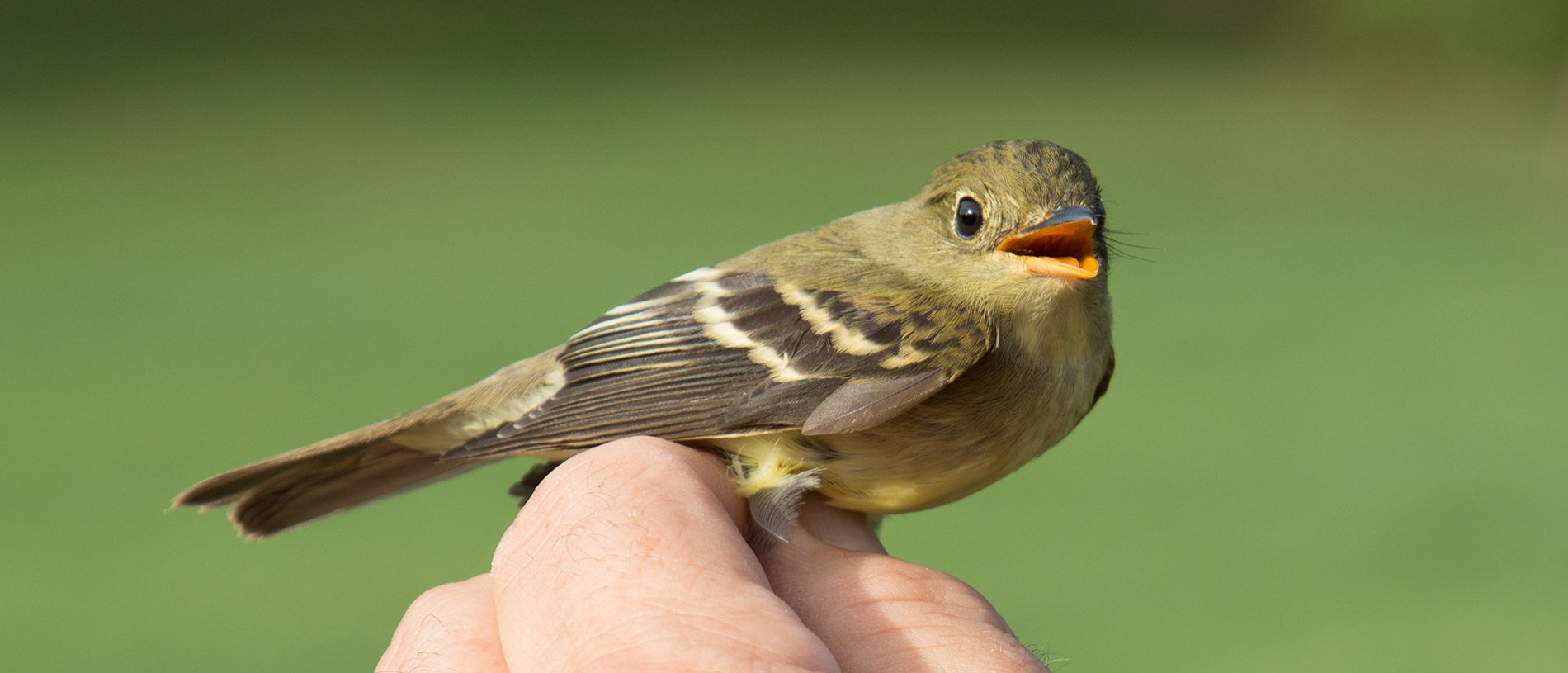In a lush, natural outdoor setting, characterized by a blurred backdrop in varying shades of green and dark green, a human hand is gently holding a small bird. The bird, a captivating mix of yellow and greenish-yellow hues, is perched with its feet nestled between the person's thumb, index, and middle fingers, of which only the tips are visible in the lower part of the image. The bird's body is oriented to the right, but it intriguingly turns its head to gaze directly into the camera. Its beak, partially open and revealing an orange interior, contrasts with its black upper mandible. The beady black eye is prominently displayed. Decorated with intricate patterns, the bird's crown flaunts olive green feathers accented by grey wisps, transitioning into a breast adorned with subtle gray lines. The wings feature an elaborate design of mustard yellow, black, and pale yellow streaks, with similar coloration extending down its tail feathers. The upper portion of the image has a slightly darker hue, adding depth to this serene, detailed capture of nature’s delicate beauty.